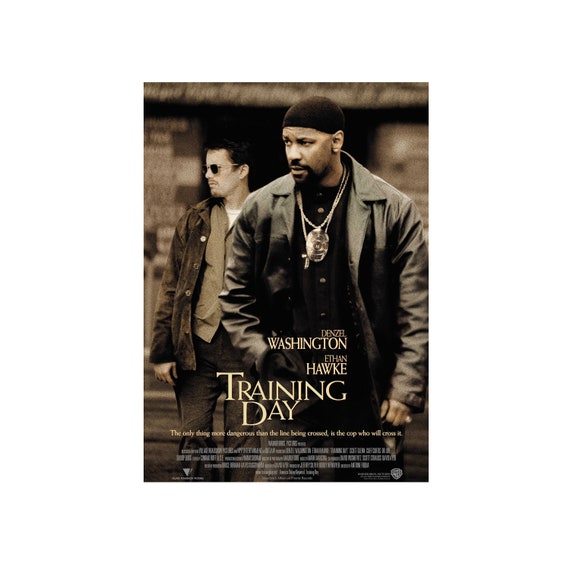The movie poster for "Training Day" features a dark, sepia-toned image with a cityscape backdrop. Dominating the forefront is Denzel Washington, facing slightly left with a stern expression. He sports a black skull cap, heavy gold chains, including a significant cross, and a police badge on a chain around his neck. His attire includes a black leather jacket over a black shirt, enhanced by his goatee and mustache. Behind him, slightly to the left, stands Ethan Hawke, looking off to the left as well. Ethan wears sunglasses and a more casual ensemble of a brown button-up jacket over a white t-shirt and blue jeans. The poster displays the actors' names in large white text at the top: "Denzel Washington" and "Ethan Hawke." Below, the title "Training Day" is prominent, accompanied by the tagline: "The only thing more dangerous than the line being crossed is the cop who will cross it." Further details about the film's production, although present, are less legible at the bottom.